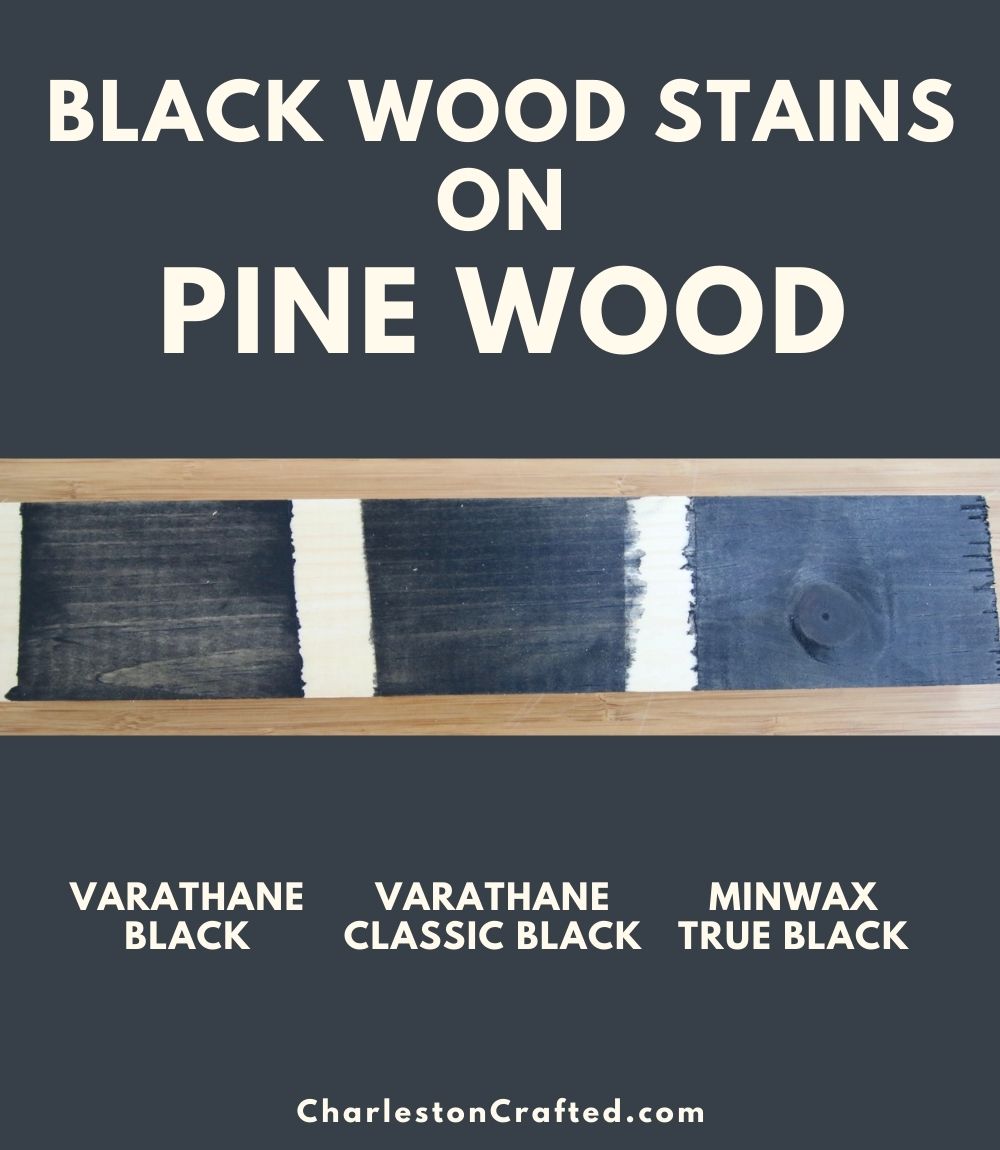The image showcases a promotional brochure page for black wood stains on pine wood, emphasizing the differences between three types of black stains. The top of the page features the title "Black Wood Stains on Pine Wood" in white lettering. Below this, a piece of lightly stained, blonde pine wood is displayed with distinct sections: on the left, the stain is lighter, it darkens somewhat in the middle, and on the right, it is the darkest. The stains are labeled as "Varathane Black," "Varathane Classic Black," and "Minwax True Black," highlighting their different intensities and hues. The wood overall displays a gradient of grays and bluish tones, with two white stripes running through the center of the black-stained sections. At the bottom, the page is marked with the website "charlestoncrafted.com" in white letters, indicating its origin. The background of the brochure shifts from dark blue at the top to dark navy blue at the bottom, giving a contrasting backdrop to the stained wood samples, making this a visually informative piece likely featured online or in a printed brochure.